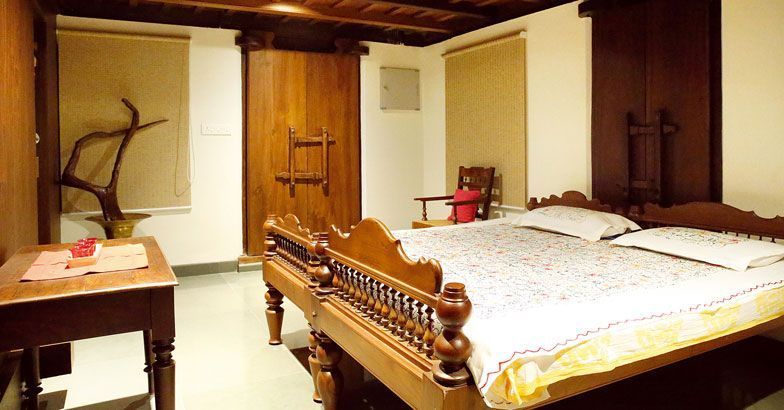This old-fashioned bedroom features two twin beds pushed together, framed by brown wooden headboards and footboards. The beds are unified by a thin white quilt adorned with faint red specks and a subtle floral pattern, alongside two flat pillows. At the bottom-left corner of the room is a wooden end table, partially covered with what appears to be a sheet of paper or fabric and some small, unidentifiable red items. Above this table, against the back wall, hangs a window with its shade drawn, in front of which stands a sculpture resembling a tree with a metal base or antler-like structure emerging from a golden basin. To the right of the bed, there's another shaded window and a brown wooden chair sporting a red pillow. The room is characterized by muted colors—primarily shades of brown, white, and beige. The backdrop includes two distinguished wooden doorways: one light brown and intricately carved and another darker mahogany door positioned directly behind the bed, giving the room a timeless and rich aesthetic.